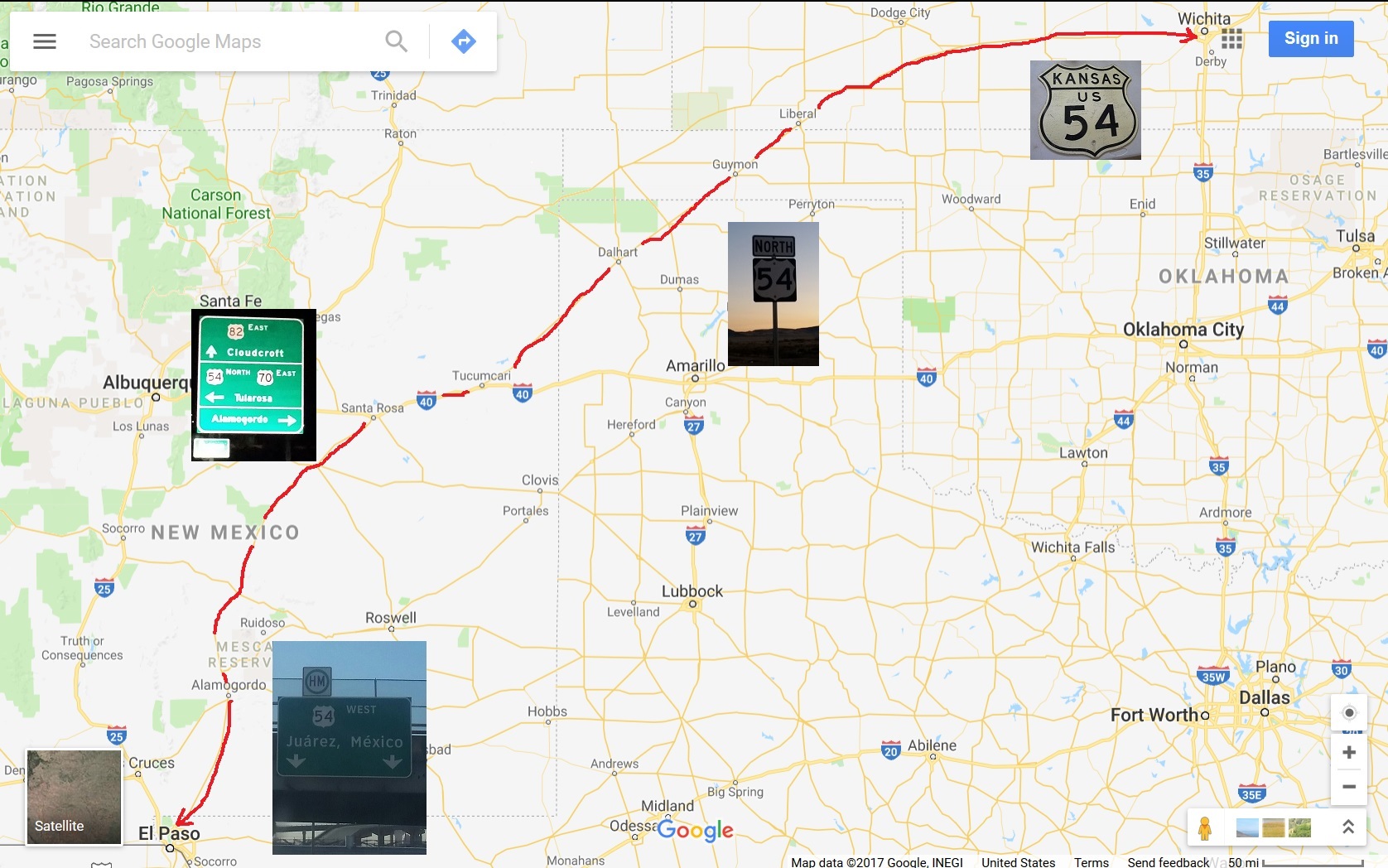This image is a detailed screenshot from the web version of Google Maps, evident by the wide screen layout and small, well-spaced icons at each corner. The map highlights a red directional path starting from El Paso, Texas and extending to Wichita, Kansas, cutting through New Mexico. This path is primarily following U.S. Route 54, a detail reinforced by multiple instances of the route number in the inset photographs. The map displays numerous yellow lines indicating roads, and green areas indicating national forests. It also labels various towns with black dots proportional to their population size. Notable cities like Oklahoma City and Amarillo, as well as significant interstate designations such as U.S. Route 40, are visible. Additionally, the lower left corner includes a satellite view insert, and superimposed images showcase road signs and landscapes encountered along the journey, including a distinctive sign against a sunset backdrop.